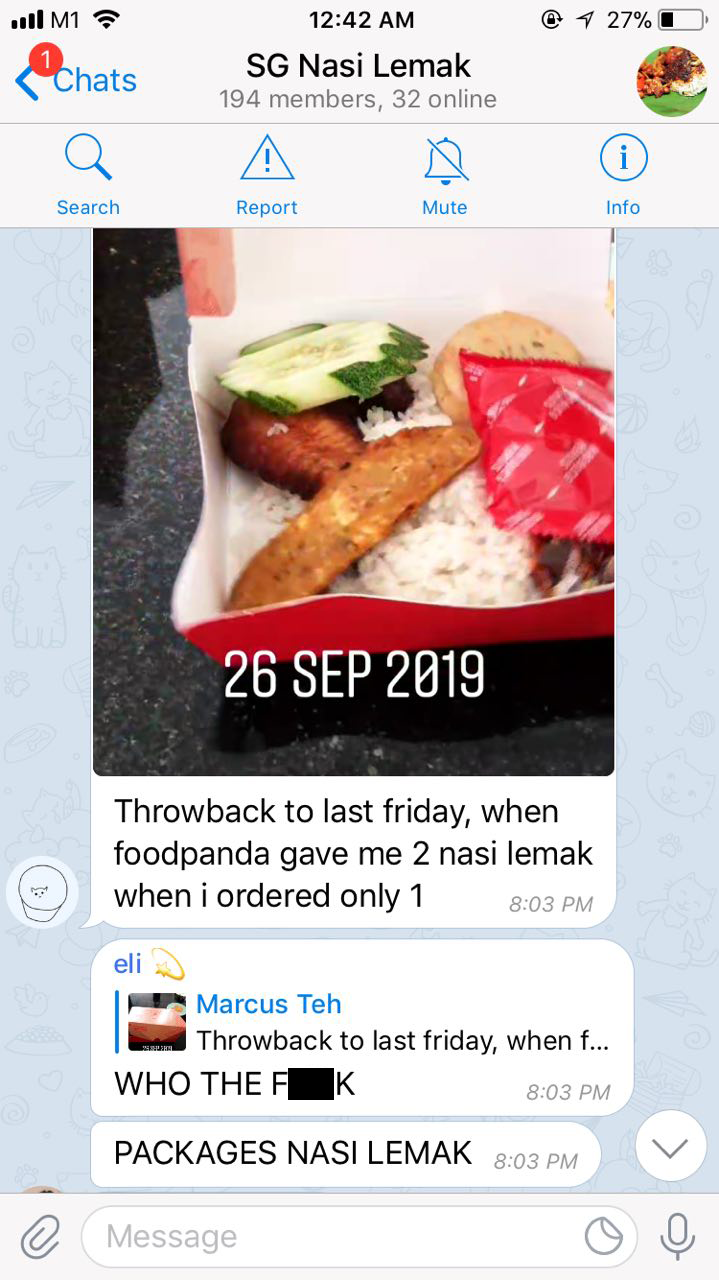This image captures a screenshot from a mobile phone, showcasing a messaging app with 27% battery life and a strong connection. The app appears to be running on the M1 model. At the top of the screen, the title "SG Nassi Lemak" is displayed prominently. Below, there is a blue chat bubble with an arrow pointing to the left and a red circle containing the number "1". 

On the right side of the screen, there's an image of food and information indicating that the group has 194 members, with 32 members currently online. The background color of the chat interface is a light gray. 

Beneath the main chat display, there are options for search, report, mute, and more info. Further down, the actual picture of the food is displayed, though slightly blurry. It features a serving of white rice, a cucumber, and what appears to be a piece of slightly burnt meat or fish. 

Overlaying the food image is the date "September 26, 2019". Below this, the caption reads: "Throwback to last Friday when Food Panda gave me two Nassi Lemak when I ordered only one." This message seems to be from someone named Eli, whose profile picture is a pink square. 

Following the message, there's a partial response from another user named Marcus T.E.H., who repeats the initial caption, implying a reply. The conversation appears to involve some frustration, as indicated by the text "who the F-U-C-K" and the term "packages Nassi Lemak," with the letters "U-C" blacked out.